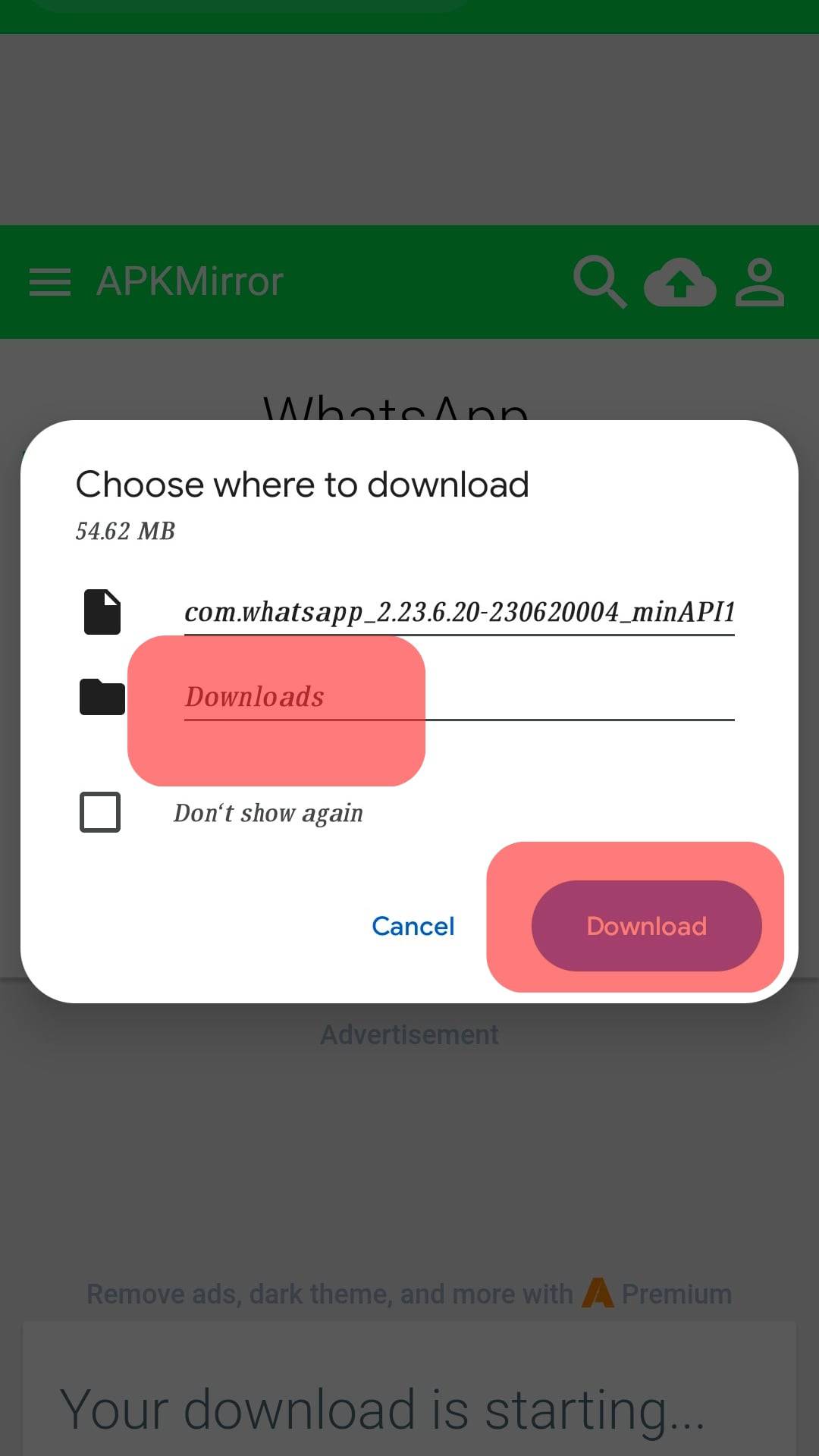This image showcases the WhatsApp application interface on a smartphone. Prominently, it features the APKMirror platform. The layout displays a distinctive green bar above a gray one, indicating the application’s identity. At the top is a search bar and an icon resembling a cloud with an upward-facing green arrow next to a generic person’s picture, emphasizing the user interface’s functional design.

Central to the image is a partially visible, white pop-up notification with "Choose where to download" at the top. This dialog instructs the user to select a destination for the download, defaulting to a folder labeled "Downloads", outlined in pink. Below this, there are options for "Don't show again" and two buttons: one for "Cancel" and another for "Download", the latter highlighted with a pink outline and purple interior, featuring the word "Download" in pink text.

Underneath the download dialog, there is an advertisement mentioning the benefits of a premium version which includes features like ad removal and dark theme. Additionally, text indicates that the download process has commenced with the message "Your download is starting."

At the very top of the image, another thin green bar stretches across without any text, adding to the visual structure of the interface.